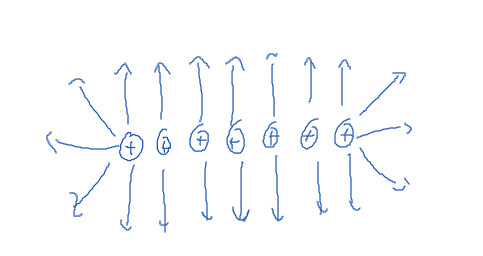The image presented is a rudimentary drawing created with MS Paint, characterized by its simplistic and amateur appearance. The drawing features a horizontal sequence of seven hand-drawn circles, each adorned with a small plus sign at its center. The circles exhibit uneven and wobbly lines, suggesting they were drawn with a computer mouse.

From each of these seven circles, arrows extend in both upward and downward directions. Additionally, the circles at both ends of the row have three extra arrows pointing towards the northeast, east, and southeast directions, forming angles of approximately 45 and 135 degrees respectively. In total, there are around 20 thin, blue pencil-stroke lines, further emphasizing the amateurish nature of the sketch. The entire composition is rendered in a monochromatic blue, adding to its simple yet intriguing visual presentation.